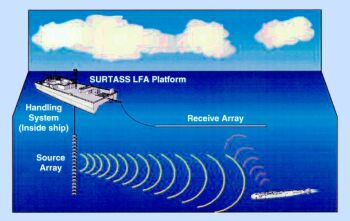This image is a highly detailed and stylized illustration, resembling both a diorama and a 2D-3D hybrid graphic, that depicts a nautical scenario involving advanced marine technology. At the top of the rectangular illustration, a flat panel represents a serene blue sky dotted with white clouds. Below this, a deep cobalt blue sea extends, on which floats a flat-decked vessel labeled "SURTASS LFA Platform." This platform, which resembles a barge with a high mast, is situated on the left side of the model.

A rope or tether descends from the ship into the underwater section, highlighted in a lighter blue to demarcate sea level. This tether is marked "Receive Array" and is connected to a vertical cylinder labeled "Handling System (Inside Ship)," which extends deep into the ocean. The ship's source array emits radar or sonar waves, depicted as concentric, expanding half-circles radiating outward from under the vessel. These waves are in detection mode, monitoring an incoming torpedo or similar object on the right side of the graphic, which in turn sends a message back to the receive array.

The entire scene is encapsulated in a light blue frame, combining vivid elements of both surface and subsurface marine technology in a single narrative tableau.